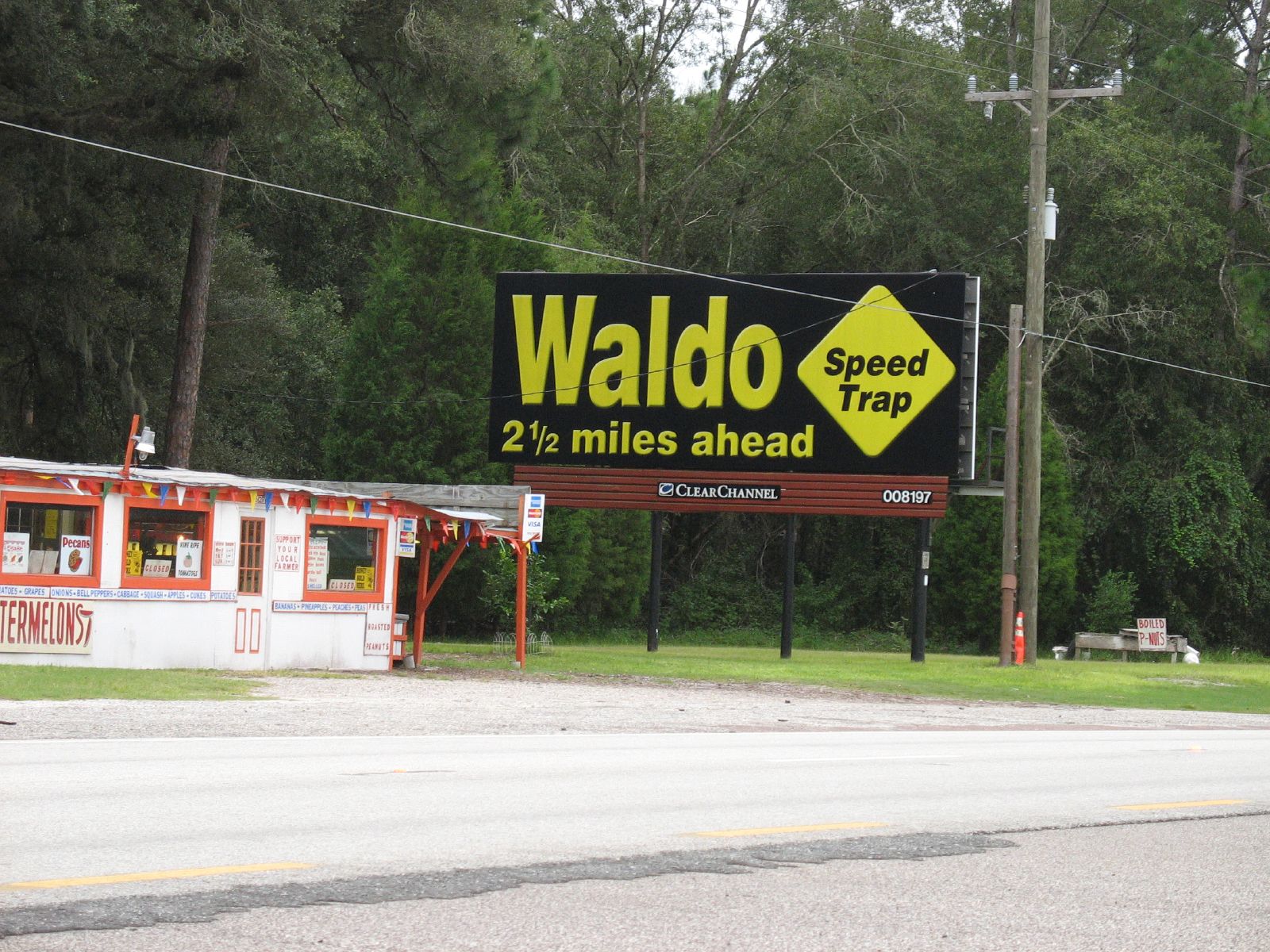The photograph captures a detailed scene of a roadside area featuring a large black billboard with bold yellow text that reads "WALDO two and a half miles ahead, SPEED TRAP," accompanied by a yellow diamond shape. The billboard, identified with the company name "Clear Channel," is placed near a highway with visible cracked concrete and yellow lines. A brown power pole with silver electrical lines stands near the billboard. Behind, thick and green large trees can be seen, providing contrast to the scene. To the side of the billboard, there is a small white building with red trimming. This roadside business, possibly a convenience store or fast food establishment, features large windows adorned with posters, and orange flags hanging from the roof. The area also includes an orange cone placed against the power pole, adding a distinct splash of color.